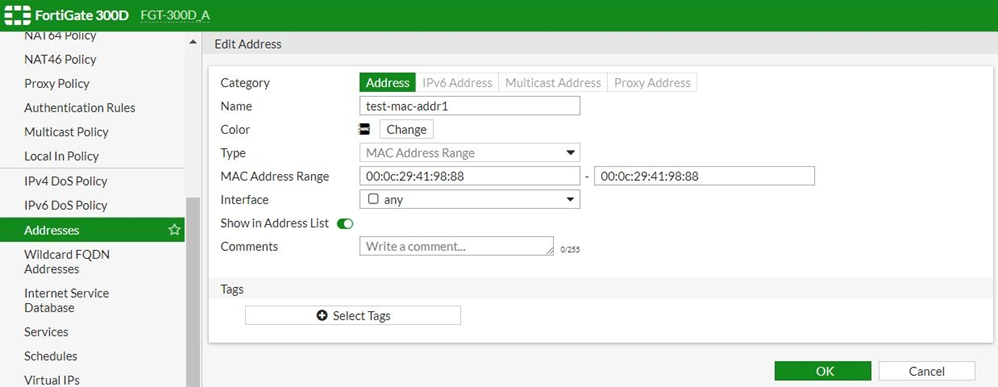This is a detailed screenshot of the ForteGate 300D website interface. In the top left corner, the site's name is displayed as "ForteGate 300D," and to its immediate right, there is an additional identifier labeled "FGT 300DA," possibly indicating the specific section or model variant being viewed. The website’s logo, situated also in the top left area, consists of multiple circles arranged in a square formation, with the central circle being green.

To the left side of the interface, a navigational panel features an array of tabs for various settings and policies. The options include: NAT64 policy, NAT46 policy, piracy policy, authentication rules, multicast policy, local and policy, IPv4 DOS policy, and addresses, which is the current selection. The addresses section allows users to edit specific addresses, as indicated by the "Edit Address" heading at the top left. The category shown is "Address" and within it, "IPv4 Address," with an individual entry labeled "Test Mac ADDR1."